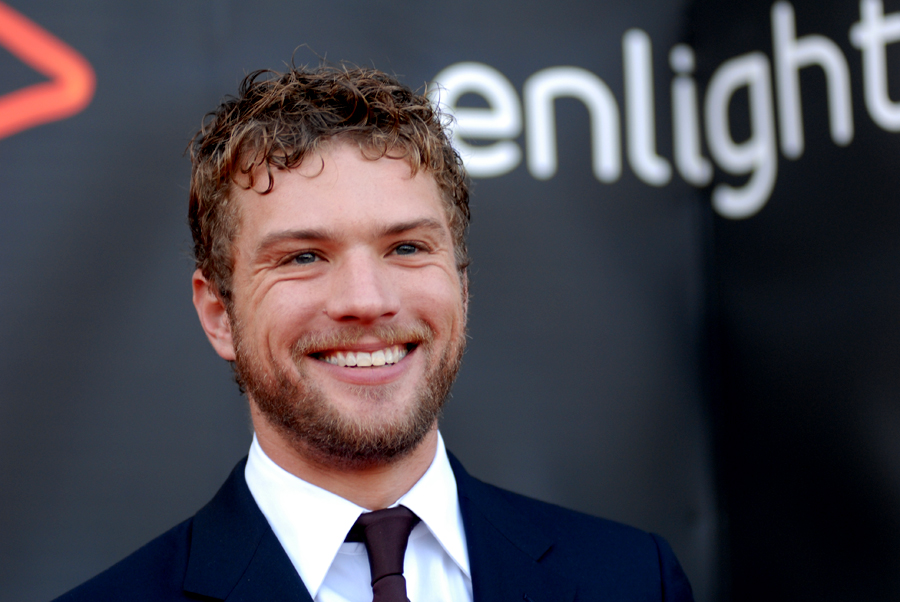This photograph features a famous actor, possibly Ryan Phillipe, standing at an event and posing for the cameras. He is smiling widely, with crinkled eyes and noticeable laugh lines, showing his teeth. The man has curly hair that appears reddish and gelled, and he sports a somewhat thick beard and mustache. He is dressed in a dark suit, which might be deep blue or black, paired with a white button-up shirt and a black tie. The background is black with thick, white lowercase text spelling "enlight" at an angle on the upper right side. There is also a red, sideways V-shaped symbol in the upper left corner of the backdrop.